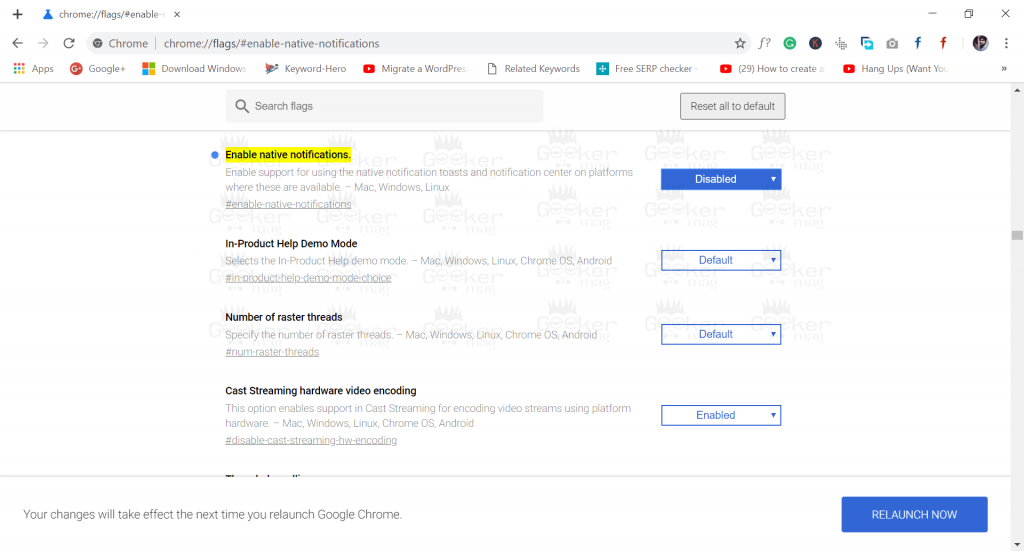This image captures a screenshot of a Google Chrome settings page, displayed as a portrait within a landscape-oriented frame, set against a stark white background. At the very top of the screenshot, an open tab labeled "Chrome Flex" is highlighted by a blue, dress-shaped icon. Below this, a horizontal white navigation bar spans the screen, featuring a back arrow, refresh button, and a gray Chrome search bar. Adjacent to these are icons along with links to various apps, including Google+ and options to download Windows.

Further down, another white bar houses a central gray search box inscribed with "Search Flags," and next to it, a gray button bordered in black and labeled "Reset All to Default." Occupying the main portion of the screenshot is an extensive white area populated with search results. The top result is denoted by a blue circle and a yellow highlight, titled "Enable Native Notifications," accompanied by a descriptive text and a blue status box indicating "Disabled." Below this entry, there is a feature labeled "In-Product Help Demo Mode," with a status set to "Default," presented in a blue box with a white center and white text.

Following this, another feature named "Number of Raster Threads" appears, also featuring a default status box. Subsequent to this, an option labeled "Cast Streaming Hardware Video Encoding" shows a status of "Enabled." At the very bottom, a gray border runs horizontally, stating that changes will take effect the next time Chrome is restarted. Finally, there is a prominent "Relaunch Now" button in blue with white text, inviting the user to apply the changes.